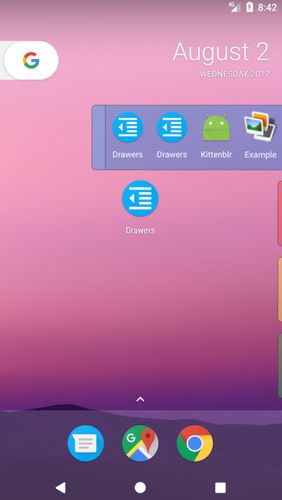This image is a screenshot from a smartphone displaying a detailed and organized home screen layout. The status bar at the top right indicates it is 8:42 AM with a full battery and a signal strength showing 2 out of 4 bars. Below this, the background transitions from light purple at the top to a darker shade at the bottom. 

On the left side, a circular icon features the multicolored Google logo (red, yellow, green, and blue) with a "G" in the center. To the right, the date is displayed: "August 2nd, Wednesday 2017."

Beneath this section, a dark purple box contains several icons: 
- On the left, there are two icons labeled "Drawers."
- To the right of these is an icon labeled "KittenBLR."
- Further to the right, another icon is labeled "Example."

Underneath this dark purple box, against the lighter purple background, another row of icons is displayed. 

At the bottom of the screen, a blue circular text icon is on the left, the Google Maps icon is centrally placed, and the Google Chrome icon is on the far right.